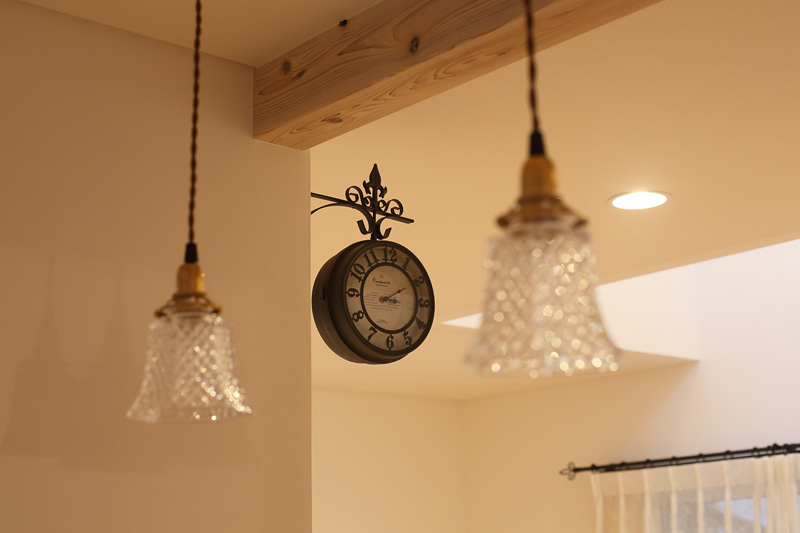The image captures the ceiling and wall of a room or hallway with an off-white ceiling accented by a large, light beige wooden beam running diagonally from the upper right towards the middle, though its full length isn't visible. Two antique-style chandeliers, hanging from dark brown or black chains with brass fixtures and glass globes, are suspended from the ceiling, but they are not lit. A round, rust-colored clock with a white or cream face, black numerals, and hands indicating ten after three is mounted on an ornate black wrought-iron bracket that juts out from the wall. Additionally, there's a recessed light embedded in the ceiling and a black curtain rod with one visible silver end, from which white sheer curtains are partially hanging.